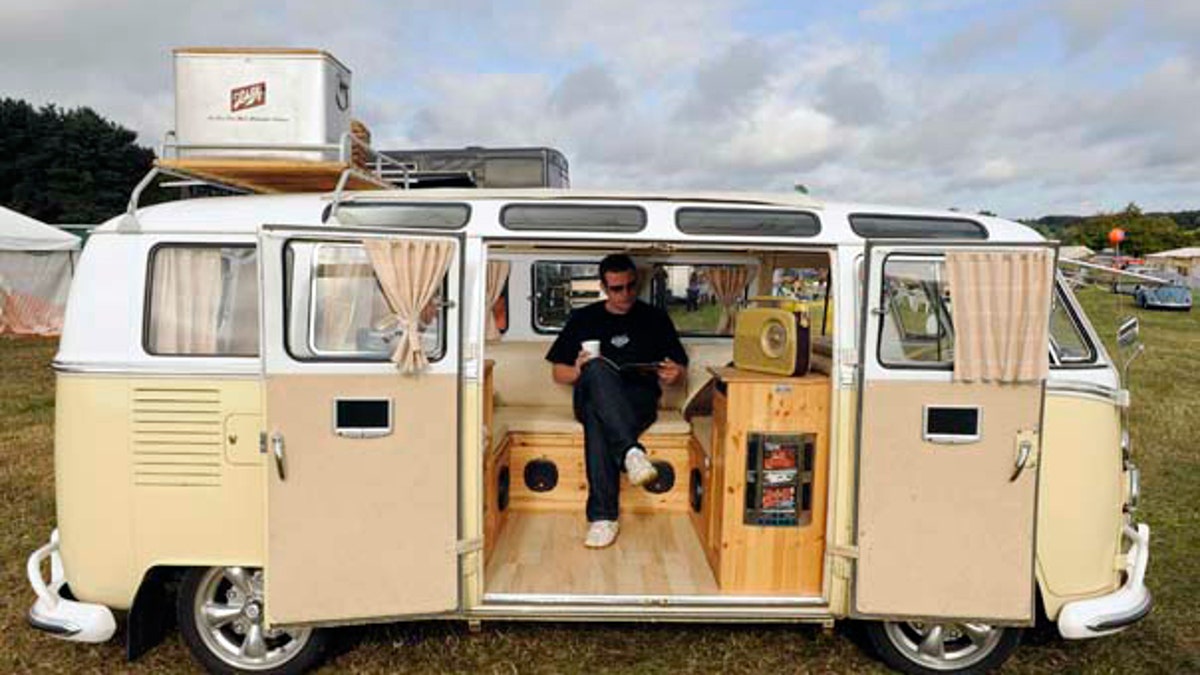The image captures a vintage van, centrally positioned in a grassy field under a partly cloudy sky with patches of blue. The van, a 1960s or 70s model, features a buff brown body with a pale beige finish and a white roof. The van's rear roof holds a white suitcase. The double doors are open, revealing the interior with wooden cabinets, a shelved radio, and seating adorned with beige cushions. A man inside, dressed in a black shirt, dark blue trousers, and white shoes, with sunglasses, is seated on a wooden bench, holding a cup of coffee and reading a magazine. He appears relaxed, suggesting the van is a recreational spot. The surrounding area includes a tent on the left side, green trees, and some distant small dwellings, hinting at a casual outdoor gathering of vintage vehicle enthusiasts.